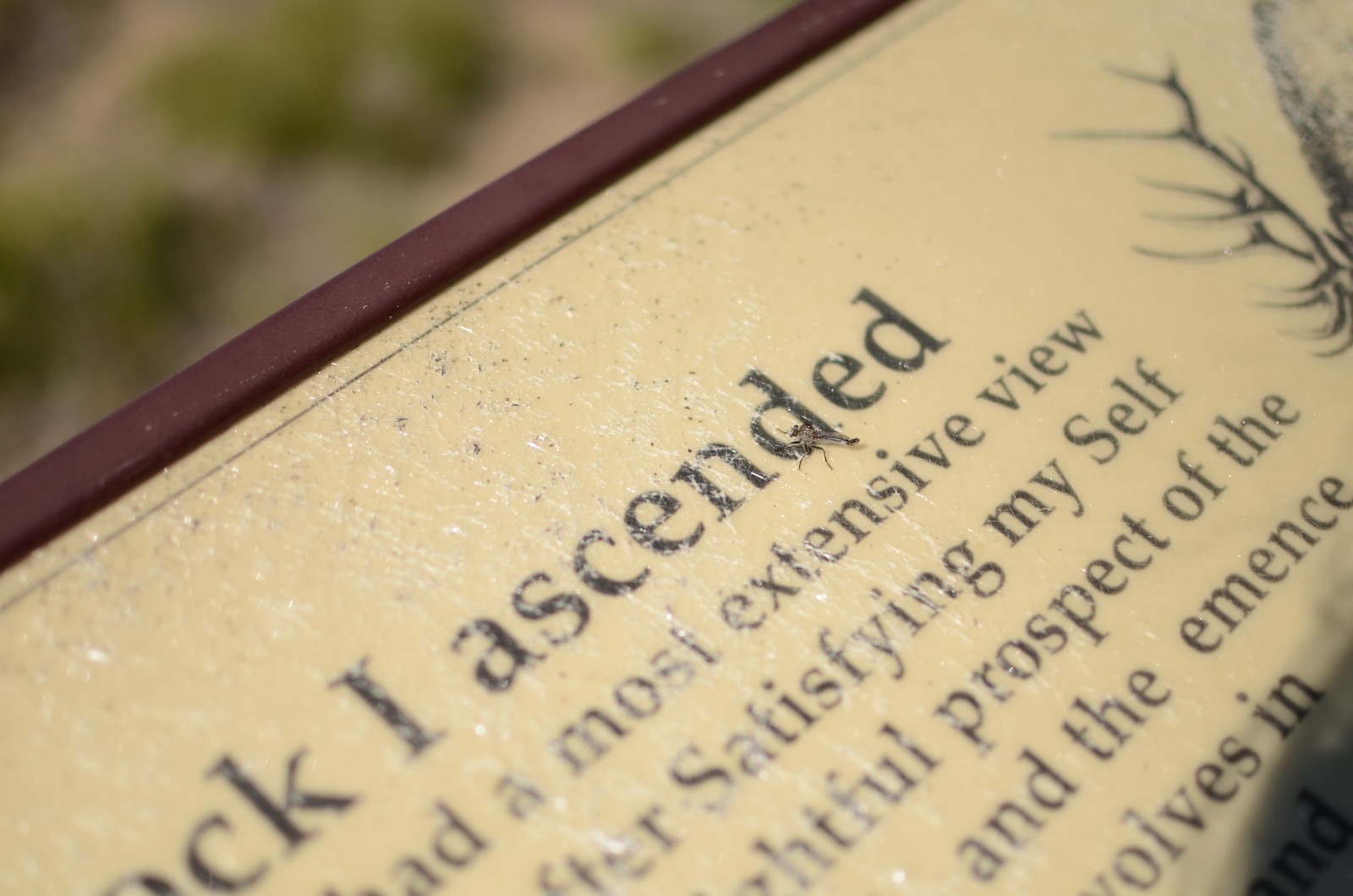This image depicts a close-up view of a weather-worn, informational sign reminiscent of those typically found in parks or natural areas. The sign, enclosed in a dark mahogany wood frame and covered with slightly cracked and yellowed plexiglass, displays black text on a cream-colored background. The most prominent and legible text at the top reads "I ascended," which seems to be part of a larger, possibly philosophical or introspective message. The rest of the visible text continues with fragments such as "a most extensive view after satisfying myself thoughtful prospect of the and the immense involves in," though its full meaning is obscure due to partial visibility. Additionally, a detailed depiction of a tree is partially visible, as well as a drawing of a deer with antlers situated to the right. Notably, a small insect, possibly a fly with a long tail and spindly legs, is perched over the first "D" in "ascended," adding an element of nature’s unpredictability to the scene.